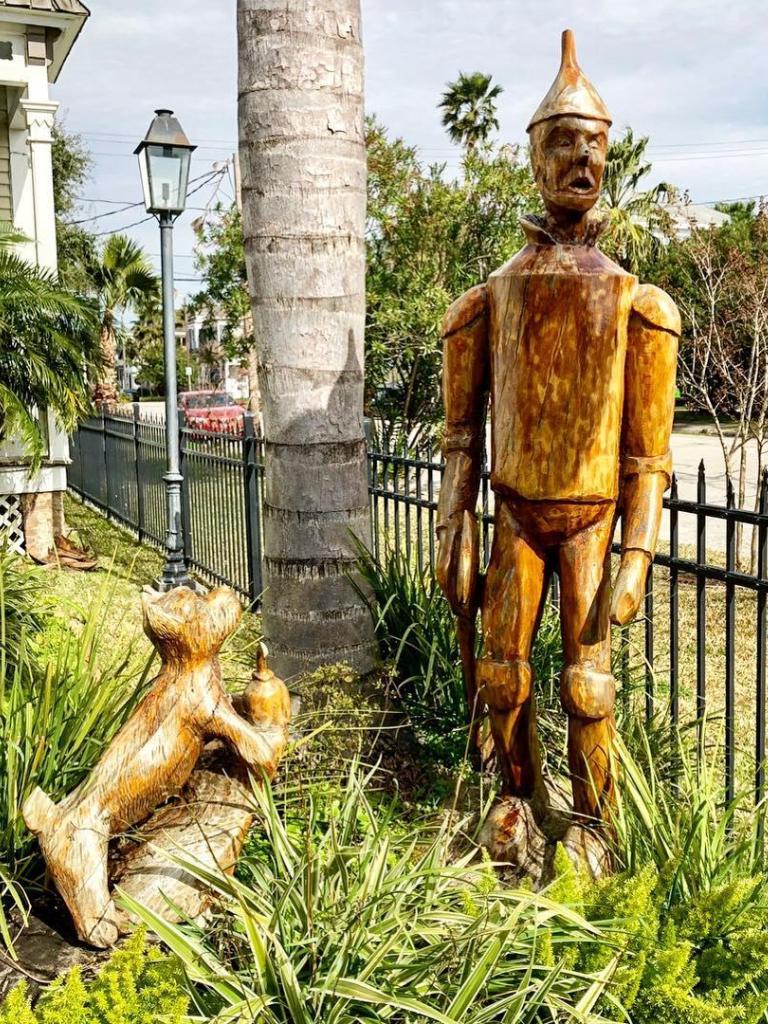In this outdoor daytime photograph, the scene prominently features a striking sculpture of the Tin Man from "The Wizard of Oz." The Tin Man, typically depicted in silver, appears rusted with a mix of golden, bronze, and brown hues. His metal body is detailed with a tin hat on his head and an instrument resembling a shovel clasped in his hand. His expression, portrayed with a downward-turned mouth, evokes a sense of melancholy. Beside him, on a raised platform, stands a golden-colored dog, likely Toto, gazing up at the Tin Man with its front paws resting on a gray log. Between the Tin Man and the dog is a tree trunk painted in gray, further accentuating the rustic aesthetic.

The background reveals additional elements of the setting: a palm tree, a red car, and a fence lining one side of the scene. There's also a lamp post near the tree, currently unlit. The scene is encased in greenery with thick grass underfoot and a broader landscape including more trees visible in the distance. The photograph, set in someone's fenced-in yard, captures the intricate details and textures of both the sculpture and its surrounding environment.